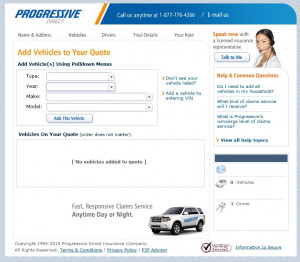**Caption:**

The image depicts a slightly blurry screenshot from the Progressive Direct website, making it difficult to read smaller font areas clearly. In the upper left-hand corner, the word "Progressive" appears slightly diagonal, slanting from the lower left to the upper right. Adjacent to this is an orange slash followed by a blue banner that reads "Call us anytime" with an additional option to email. 

On the right-hand side of the banner, there is an image of a woman with shoulder-length brown hair pulled back in a ponytail, wearing a headset on her right ear with the microphone extending to her mouth. There's a link to speak to her for assistance. 

On the left-hand side, an orange section offers the ability to add vehicles to your quote, requiring details such as type, year, make, and model. Additional options on the page include "Help" and "Common Questions" as well as "Vehicles on your Quote."

Toward the bottom left, there is a statement proclaiming "Fast responsive claim service anytime day or night," accompanied by an image of a Ford SUV with the word "Progressive" written in blue on the driver-side door panel.